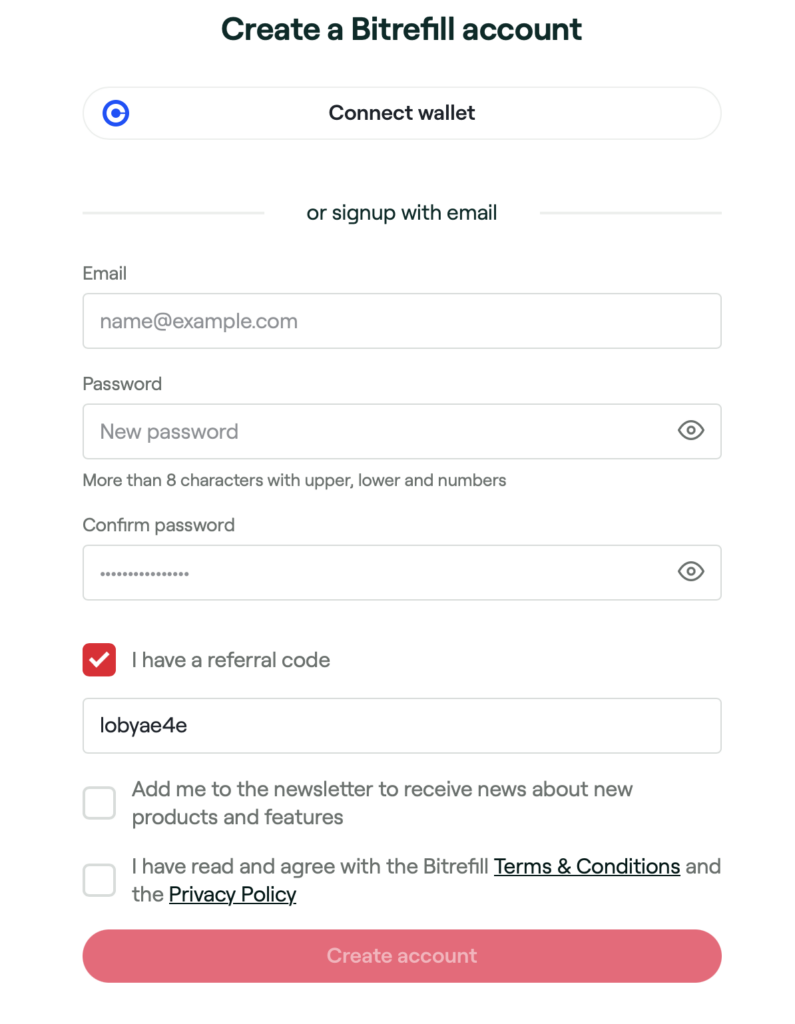The image features a user interface for signing up for a "Create a Bit Refill Account" on a website. The background is white, and the text is primarily black. At the top, there's a bold heading that says "Create a Bit Refill Account," spelled out as "B-I-T-R-E-F-I-L-L Account." Below this heading, a prominent blue circle outlined in gray with the letter "C" inside is positioned on the left side. Adjacent to this icon is a wide button stretching across the page with the text "Connect Wallet."

Beneath the button, there's a gray horizontal line that is interrupted in the center by the phrase "or sign up with e-mail," which is also in gray lettering. Below this separator, users are prompted to enter their email details. The first field is labeled "E-mail," with placeholder text "name@example.com." The subsequent field is for the user's password, with the placeholder "new password" and an eye icon next to it, indicating the option to view the entered password. There are additional guidelines below the password field, advising the user to create a password with "more than eight characters, including uppercase and lowercase letters, and numbers."

Further down is a section where users can indicate if they have a referral code, marked by a black checkbox with a white check inside. In this box, a sample referral code "L-O-B-Y-A-E-4-E" is displayed. The form also includes two optional checkboxes: one for subscribing to the newsletter to receive updates on new products and features, and another for agreeing to the terms, conditions, and privacy policies. Neither of these checkboxes are selected by default.

Finally, at the bottom of the form, there is a distinctive red button labeled "Create Account," inviting users to complete the sign-up process.